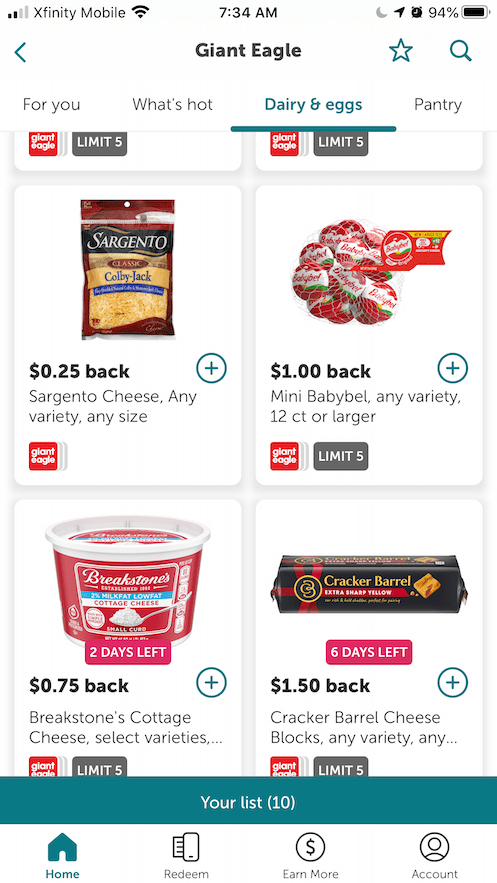This screenshot of an iPhone page shows various details prominently. At the top left corner, the network provider is displayed as Xfinity Mobile along with the signal strength indicator. Centrally at the top, the time is noted as 7:34 AM. Listed below are several items: Sargento cheese of any variety and size, mini or larger Babybel cheese of any variety, selections from Gel City, a range of Brickstone cottage cheeses of select varieties, and an assortment of Cracker Barrel cheeses.